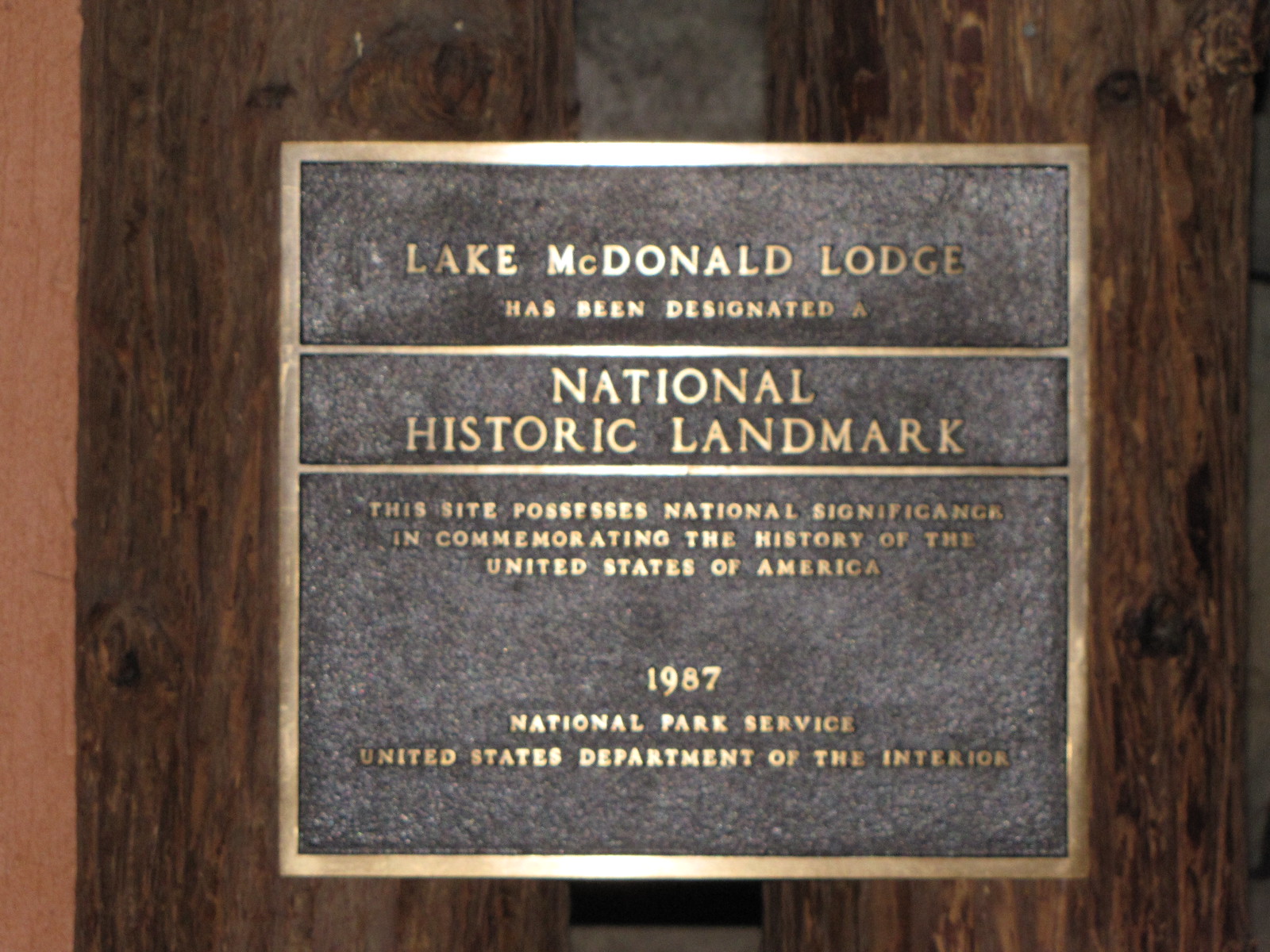The image features a dark gray, square metal sign with a gold-colored border, affixed to a backdrop of dark wooden boards. The sign reads in all capital letters, "LAKE MCDONALD LODGE" at the top, followed by "HAS BEEN DESIGNATED A" in smaller print. Below a horizontal gold line, it continues, "NATIONAL HISTORIC LANDMARK," with another gold line beneath. The text, in a serif font, states, "THIS SITE POSSESSES NATIONAL SIGNIFICANCE IN COMMEMORATING THE HISTORY OF THE UNITED STATES OF AMERICA." The inscription is followed by "1987," "NATIONAL PARK SERVICE," and "UNITED STATES DEPARTMENT OF THE INTERIOR." A prominent feature is the bronze-colored text and border, set against the mottled dark gray background, giving the sign a formal and dignified appearance. To the left of the sign, a light beige strip runs vertically, possibly part of the surrounding structure. The sign is mounted against a rough, pebbled black surface, enhancing its historical gravitas.